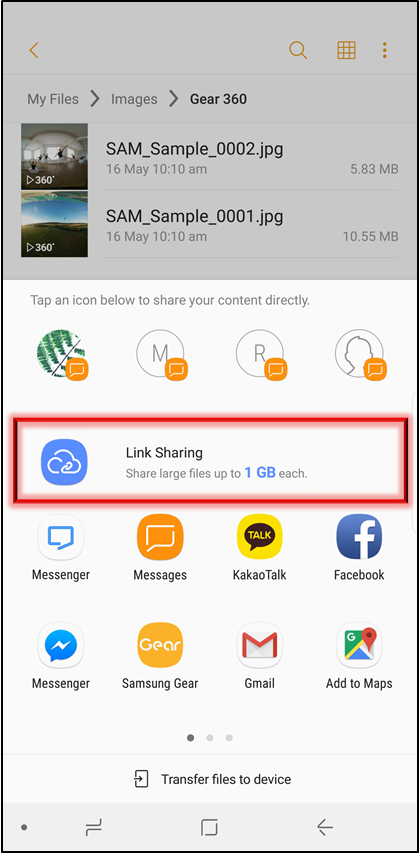Sure, here's a cleaned-up and detailed caption based on the description provided:

---

Screenshot of a smartphone interface displaying a file-sharing screen. At the top, there is a grayed-out search bar with a search icon, followed by the text "My Files > Images > Gear 360". Below, two image files are listed: "Sam_sample_002.jpg" (dated 16 May, 10:10 AM, 5.83 MB) and "Sam_sample_001.jpg" (dated 16 May, 10:10 AM, 10.55 MB).

The primary focus is on the sharing options. At the top of this section, in gray text, it says, "Tap an icon below to share your content directly." Four main sharing icons follow: one resembling a leaf, one with an "M", one with an "R", and one depicting the outline of a person. A red box highlights this region, indicating it as the current focus.

Below these options, a blue icon featuring a white cloud offers "Link Sharing", allowing the user to share large files up to one gigabyte each. Additionally, there are eight other sharing icons listed: Messenger, Messages, KakaoTalk, Facebook Messenger, Samsung Gear, Gmail, Add to Maps.

At the bottom of the screen, there's an option labeled "Transfer files to device". The interface concludes with a light gray bar housing additional navigation menu and option buttons.